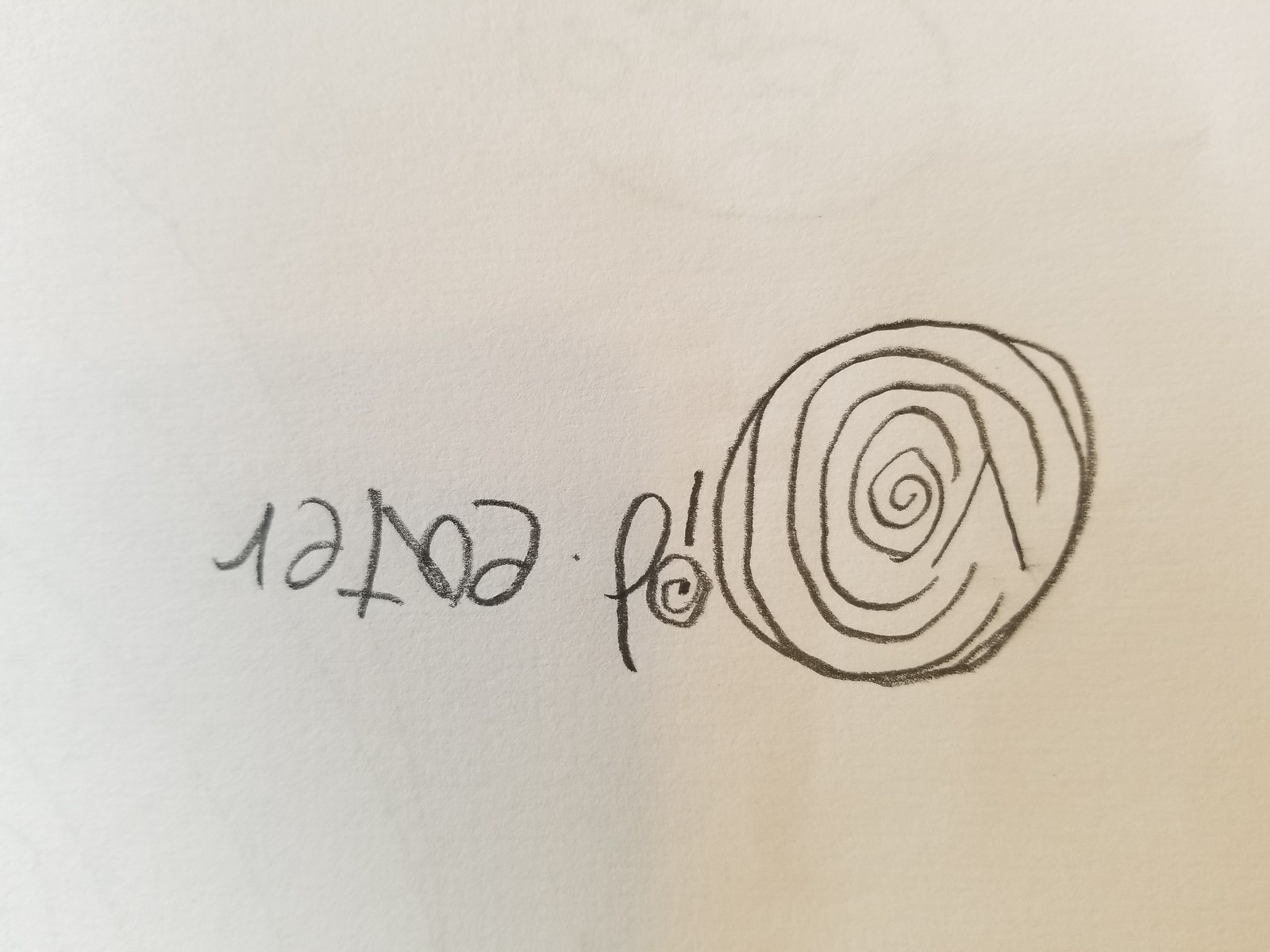The photograph features a slightly off-white piece of paper with a mixture of doodles and writing. Dominating the image is a crude, hand-drawn spiral design made up of several concentric, imperfect circles, resembling a child’s drawing. The larger outer circles gradually decrease in size towards a tiny central circle, forming a spiraling pattern. Above this spiral, there appears to be a faint remnant of another circle that has been partially erased. Positioned next to this design, but inverted, is a collection of letters and symbols which, when read correctly, spell "add eater." The letters are disjointed, with some flipped in different directions: an arrow pointing up, a backward 'E,' an upside-down 'T,' a backward 'A,' another backward 'E,' and a properly oriented 'P,' followed by an '@' symbol. The dot of the 'i' in "id eater" (when viewed upside down) also features a miniature version of the spiral pattern. The overall impression is that of an intricately chaotic doodle, combining both playful art and scattered text on a single canvas.